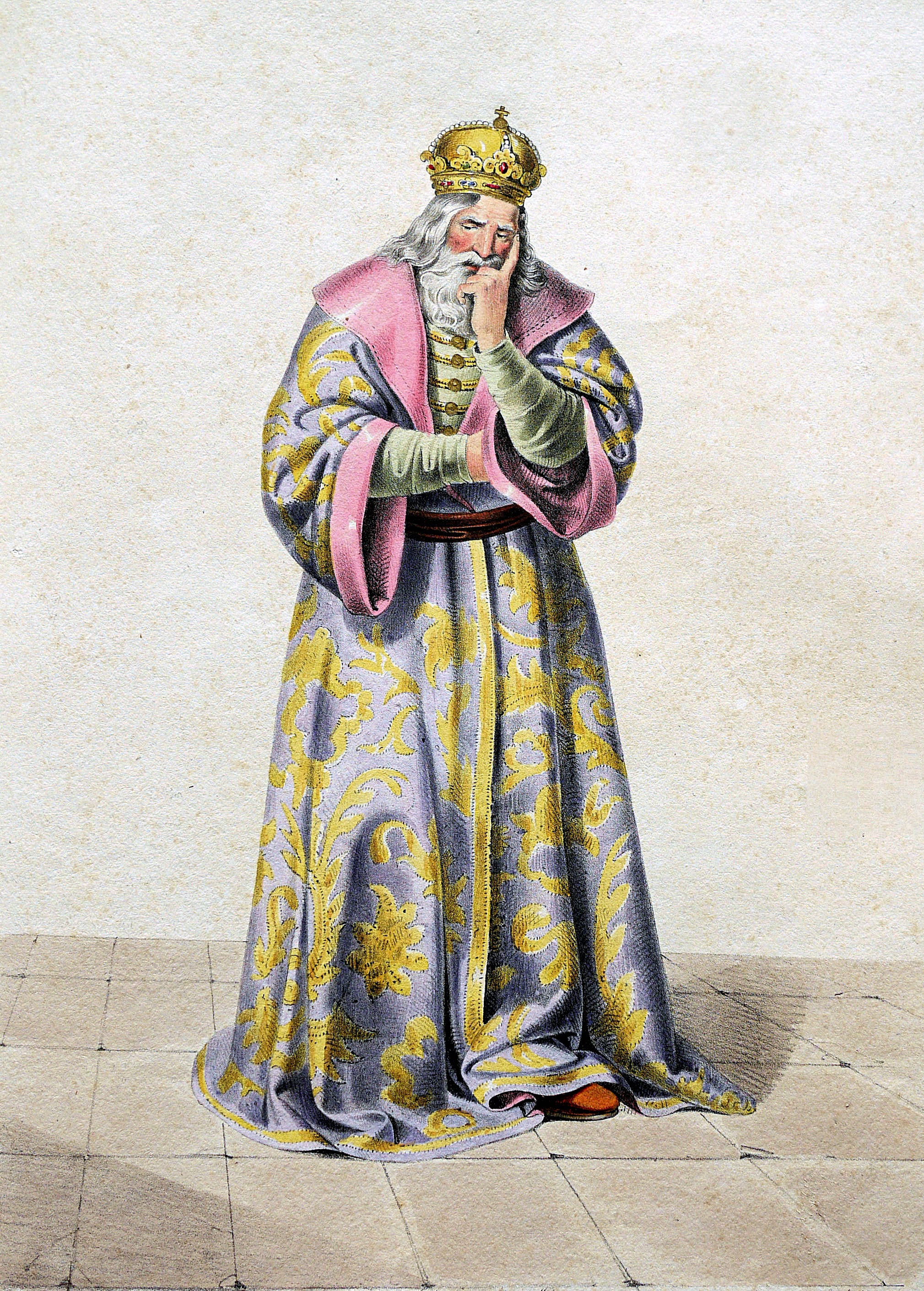This artwork, titled "Geza II," is a color lithograph from 1828 by Josef Kriehuber. It depicts an elderly king of light-skinned descent, standing on a tiled stone floor that is plain and rectangular. The background is an off-white, possibly a representation of a wall. The king is adorned in an ornate, full-length robe of bluish-purple hue with intricate gold designs resembling leaves and plants. The robe features a pink satin collar and cuffs. His long white hair, slightly curled, cascades over his ears, and he also has a long white beard and mustache, along with white eyebrows. The king wears a rounded gold crown embellished with fleur-de-lis motifs and a cross on top, set with jewels along the border. He is posed with bent elbows, his left hand resting against his face with his index finger extended along his cheek, gazing contemplatively down to the lower left. Part of his brown shoe peeks out from beneath his lavish robe.